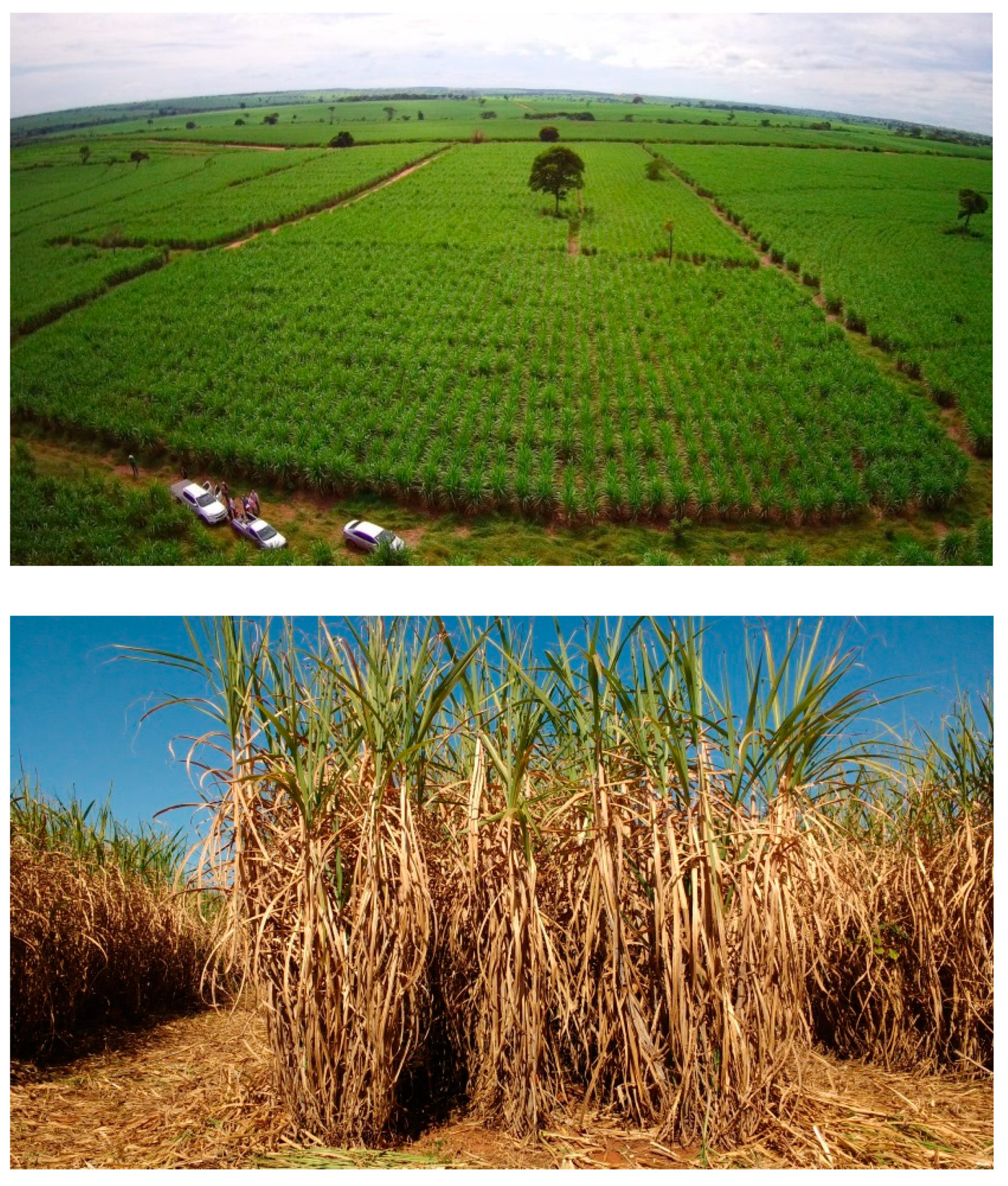The image consists of two juxtaposed photographs of farmland, with the top one displaying an aerial view and the bottom one taken from ground level. The aerial shot on top reveals an expansive area segmented into numerous green fields, with some centrally located trees unexpectedly remaining amidst the farmland. Three different vehicles—a truck, an SUV, and a car—are parked at the front, with people seen alighting from them, possibly to inspect or work on the crops. The horizon features a backdrop of hills or mountains under a cloudy yet sunny sky with patches of blue. The lower photograph focuses on the crops up-close, showcasing rows of green plants emerging from a dry, brownish base that resembles bark. The precise nature of the crop remains unclear but suggests characteristics akin to pineapple tops or some type of grass. The scene is enriched by the varied hues of brown, light brown, green, dark green, black, and white, accentuating the daytime setting in this idyllic outdoor landscape.